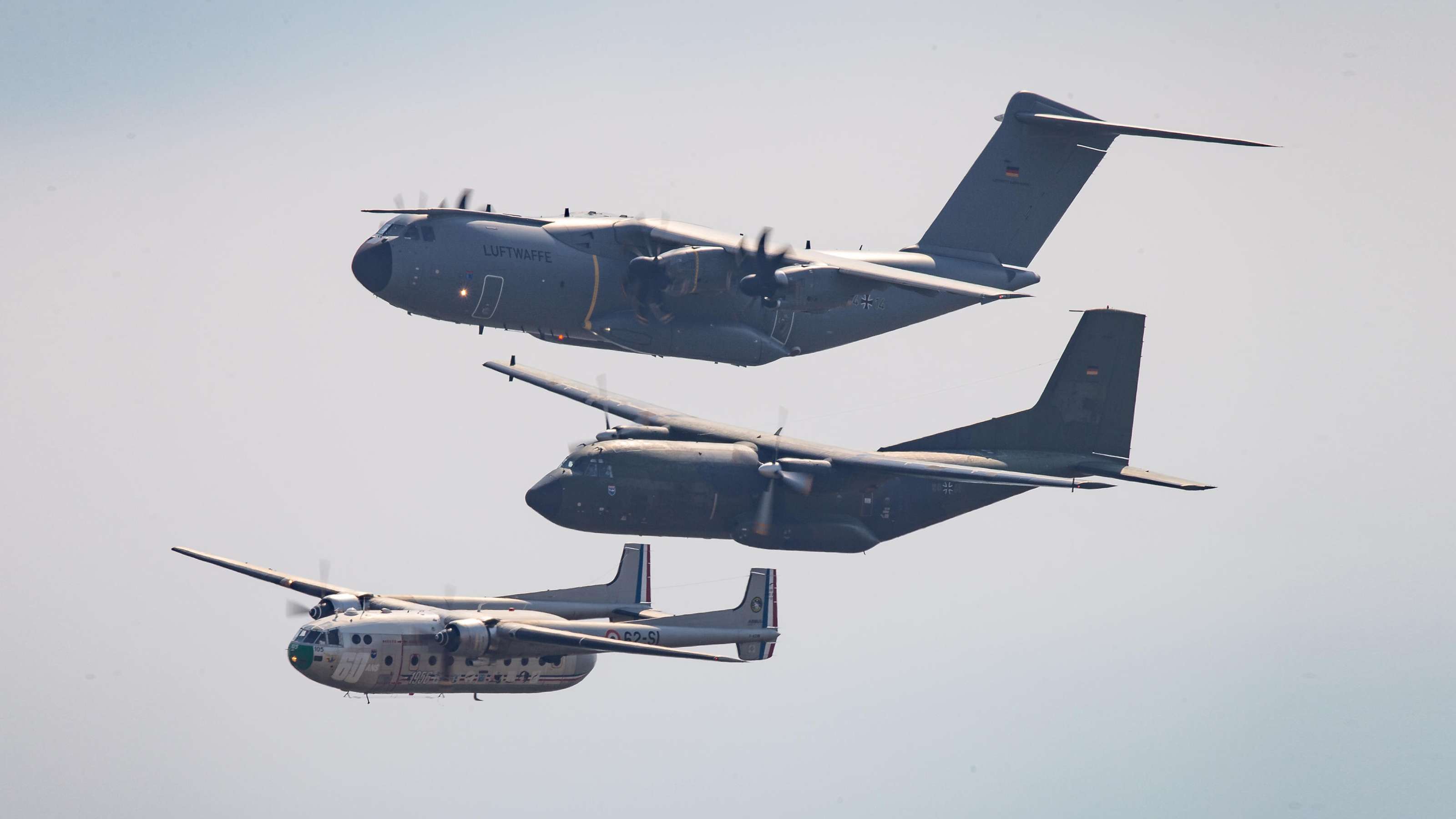The image showcases three large World War II-era turboprop planes flying in formation against a light blue, almost white sky. The uppermost aircraft features a dark gray nose, a silver body, overhead wings, and four propellers. It sports a squarish tail and looks built to carry heavy loads. This plane's significant girth suggests it could transport heavy equipment or vehicles. The central aircraft, positioned more to the right, mirrors the upper plane’s overhead wing design but is distinguished by a shorter nose and a more typical single tail. It has two propellers, also indicative of a robust, transport-class airplane. The lowest plane in the formation features twin tails, a lighter metallic, almost aluminum body, and two engines. With a fuselage that appears to have multiple window openings, this plane likely serves transport purposes as well. The formation's composition and background hint at a flyby event, given the historical nature of these aircraft. The light blue sky, devoid of distinct clouds, enhances the scene, making it difficult to discern if the planes were superimposed or captured in an actual aerial maneuver.